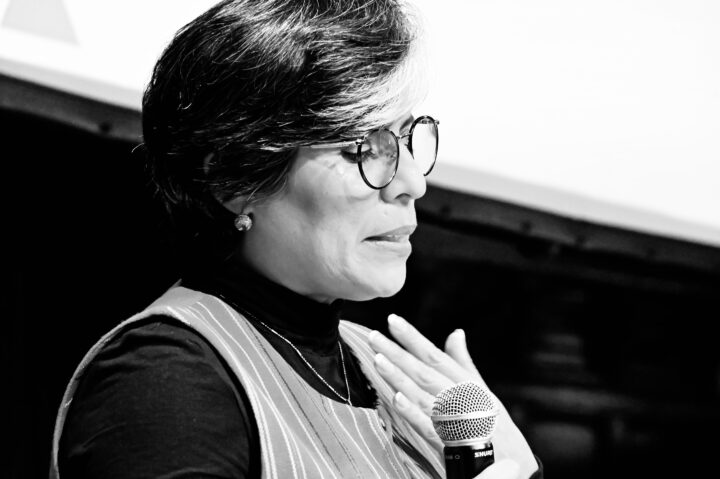This professional black and white photograph captures a side view of a middle-aged woman, appearing to be in her late 50s, from her shoulders up. She has short, salt-and-pepper hair, and is adorned with round glasses and a single earring on her right ear. She is wearing a vertically striped, sleeveless jumpsuit over a dark turtleneck shirt, and a necklace can be seen around her neck. Her left hand, displaying a well-manicured square-round French manicure, rests on her left shoulder, while her right hand holds a microphone, its metallic head partially visible near her mouth. Her expression is serious and somewhat sad, as she gazes downward. In the blurry background, there is a dark structure topped with a lighter roof, suggesting some type of building or possibly a screen. The entire scene is depicted in striking black and white, adding to the somber mood of the photograph.